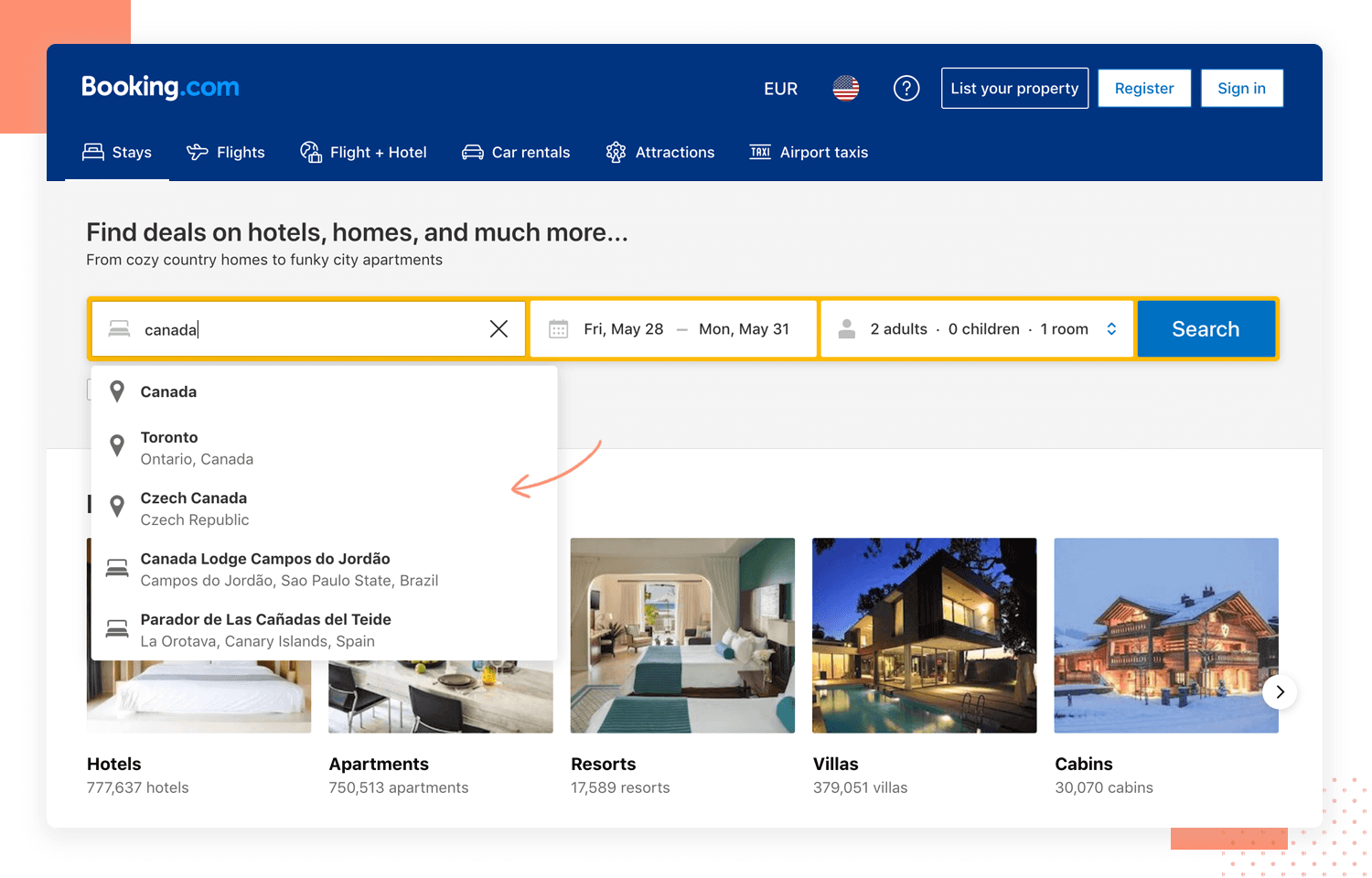Caption: 

The Screenshot of a Booking.com Webpage Showcasing Travel Options from Canada
 
At the top of the Booking.com webpage, a distinct dark blue banner spans the entire width of the screen, accented by a terracotta-colored patch. The site's logo, "Booking.com," is prominently displayed, with "Booking" rendered in white against the dark blue background and ".com" in bold blue, creating a visual contrast. To the right of the logo, various options are visible, including a dropdown for currency (EUR), a circular icon of the American flag, a question mark for help, a rectangular button inviting users to "List Your Property," and white buttons labeled "Register" and "Sign In."

Beneath the primary banner, navigation options are defined by icons: a bed for "Stays," an airplane for "Flights," a suitcase and globe for "Flight + Hotel," a car for "Car Rentals," a Ferris wheel for "Attractions," and a taxi sign for "Airport Taxis." These icons allow users to explore different services the website offers.

Mainly focused on finding deals, the core section reads: "Find deals for hotels, homes, and much more," with a sub-caption promoting "cozy country homes to funky city apartments." The user-selected settings are showcased in respective boxes: the location is set to "Canada," the dates from "Friday, May 28th to Monday, May 31st," and accommodation for "two adults, zero children, in one room." A blue "Search" button in white text is placed to the right for executing the query.

The search results display an assortment of locations associated with 'Canada,' including:
1. Toronto, Ontario, Canada
2. Česká Kanada in Czech Republic
3. Canada Lodge in Campos do Jordão, São Paulo State, Brazil
4. Parador-Lecas-Cañadas-Del-Tíde on La Orotava Volcanaria Island, Spain

Additional photos and advertising for various accommodations like hotels, apartments, resorts, villas, and cabins can be seen at the bottom of the page, presenting diverse lodging options globally.